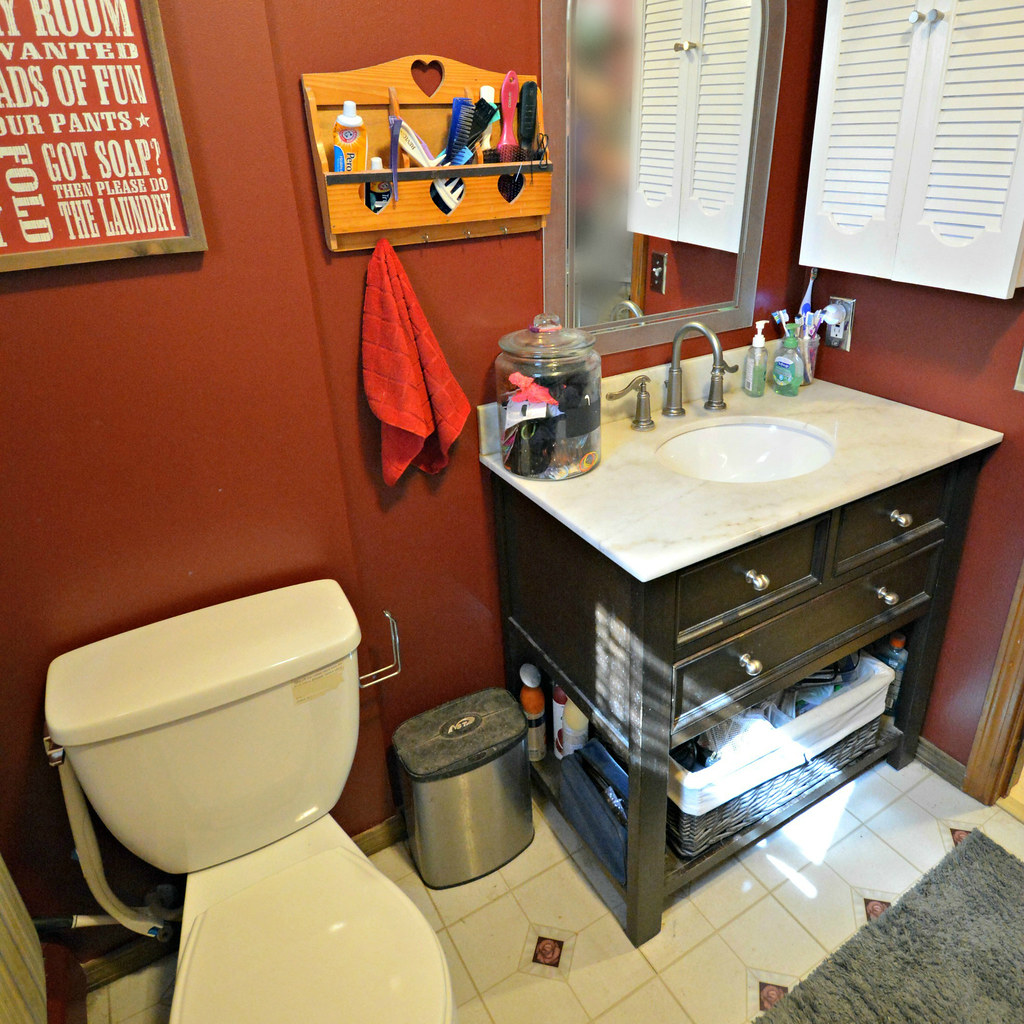This indoor photograph captures a cozy bathroom with rich brown walls, showcasing two adjoining walls. On the right side of the image, there is a wall-mounted cabinet featuring louvered doors with gleaming metal handles. Below the cabinet, a wooden sink vanity stands, its base open to reveal three drawers: one large central drawer and two smaller side drawers. A clear glass jar containing a comb sits neatly on the vanity.

Mounted on the wall above the vanity is a rack that holds a tube of toothpaste and a couple of combs, with hooks beneath it from which a red washcloth hangs. Beside the vanity, a white toilet is stationed, above which a whimsical sign reads in white letters against a red background: "Room Wanted, Loads of Fun, Your Pants, Fold, Got Soap, Turn, Please Do the Laundry."

On the floor, a small metal trash can with a black lid is placed, complementing a nearby empty hook intended for holding toilet paper. The flooring consists of white tiles punctuated by a gray rug, with a striking black or reddish design at the center that harmonizes with the brown walls.